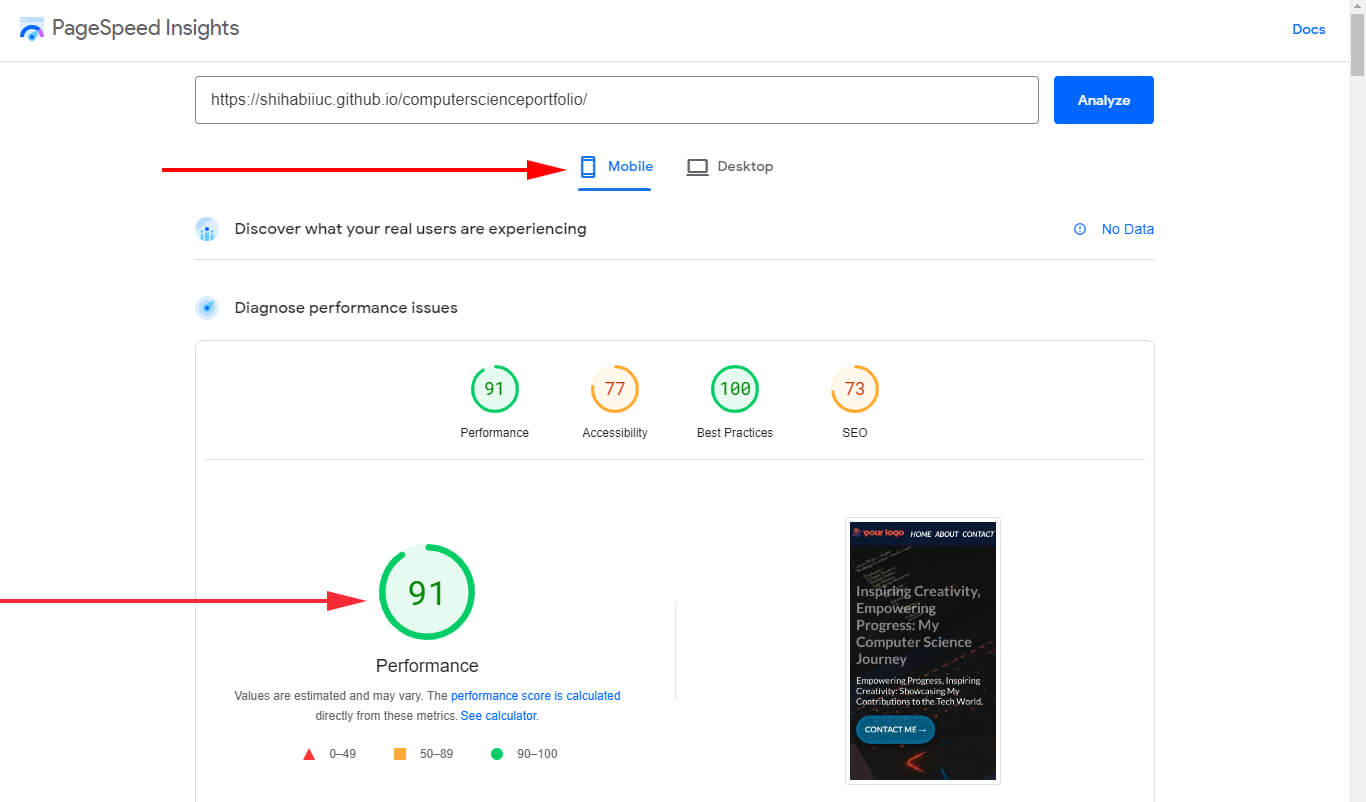The image displays a webpage for testing website speed, featured on Google’s PageSpeed Insights tool. The header reads "PageSpeed Insights" with a prominent blue and purple speed dial situated prominently beneath it. The webpage has a clean, white background.

On the upper-right corner, there is a clickable link labeled "Docs." The URL bar indicates a site is ready for analysis, accompanied by a blue "Analyze" button to its right.

A long red arrow points to a tab labeled "Mobile," which is highlighted in blue, indicating the current focus. Adjacent to this, the "Desktop" tab is highlighted in gray. Beneath these tabs, a message reads, "Discover what your real users are experiencing." However, the data section is currently blank and displays "No data."

Further down, the section “Diagnose performance issues” lists several scores:
- Performance is highlighted with a score of 91%, encapsulated within a green circle.
- Accessibility is shown with a score of 77%, presented in an orange circle.
- Best Practices is listed at a perfect score of 100%, in green font.
- SEO is rated at 73, noted in an orange circle.

Another red arrow points back to the "Performance" score, reiterating its 91% value in green. A disclaimer at the end of the section reads, "Values are estimated and may vary. The performance score is calculated."